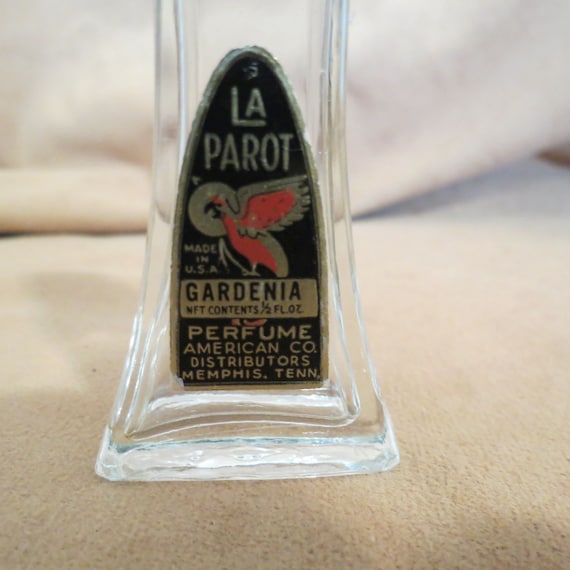This detailed image showcases a close-up photograph of an empty, clear glass perfume bottle resting on a beige surface, likely a pair of towels or a cushion. The uniquely shaped bottle features a wide base that tapers towards the top with a slight bend. Positioned slightly to the left in the photo, the bottle carries a distinct black label in an oval-like shape, with the bottom of the oval being flat. The label is adorned with silver and gold writing, reading "La Perret" at the top. Below this, there is an image of a parrot, depicted in red, gold, and hints of brown and green, encircled by additional green detailing. Beneath the parrot picture, the label states: "Made in the USA, Gardenia, Net Contents, 1 1/2 fluid ounce, Perfume, American Co. Distributors, Memphis, Tennessee." The bottle’s extreme clarity and unique design are accentuated by the soft, unfocused background, making the intricate details of the label and the glass bottle itself the focal points of the image.